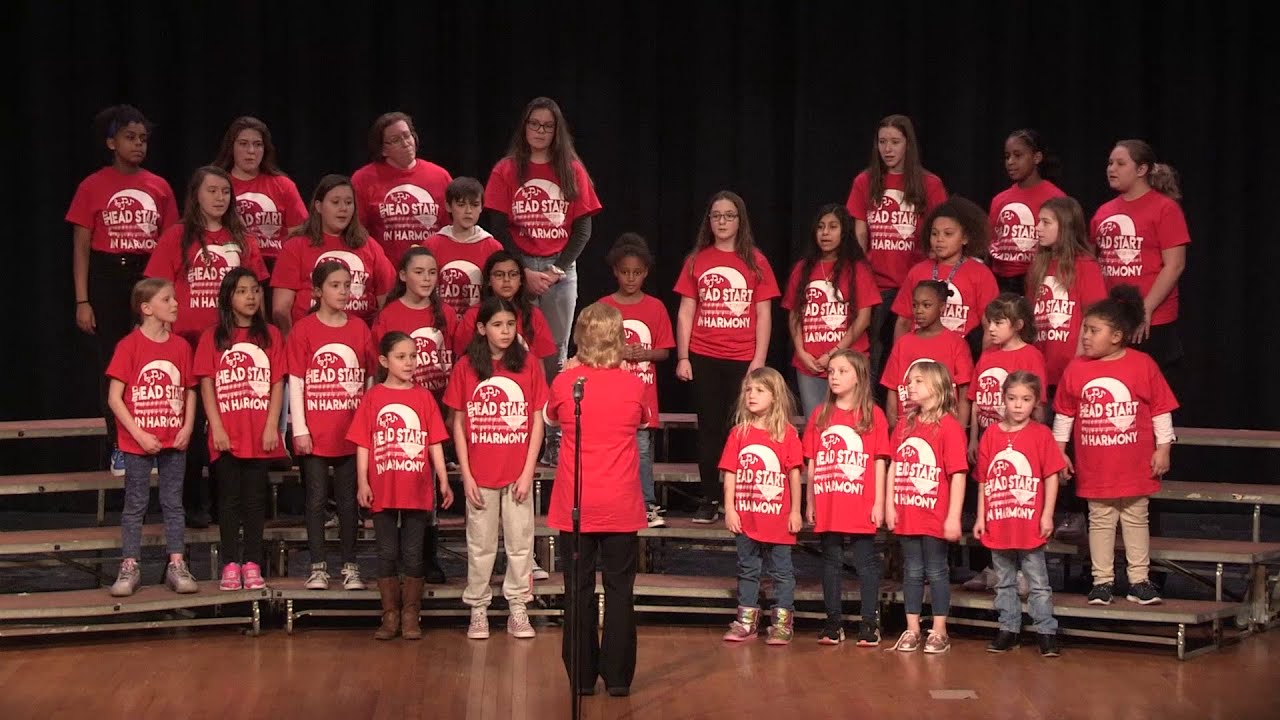The image depicts a diverse group of children from kindergarten to middle school standing on silver metal risers, participating in a choir performance. The children, all girls, are dressed in red t-shirts featuring the text "Head Start in Harmony," and are wearing various types of pants and shoes in colors such as blue, black, tan, pink, brown, and white. In front of the children, an older female conductor with long blonde hair, dressed in a red top and black slacks, stands on a wooden floor, her back to the camera as she directs them. The scene is set against a black curtain backdrop, with a microphone stand positioned to one side, emphasizing the organized yet vibrant atmosphere of a school choir performance.